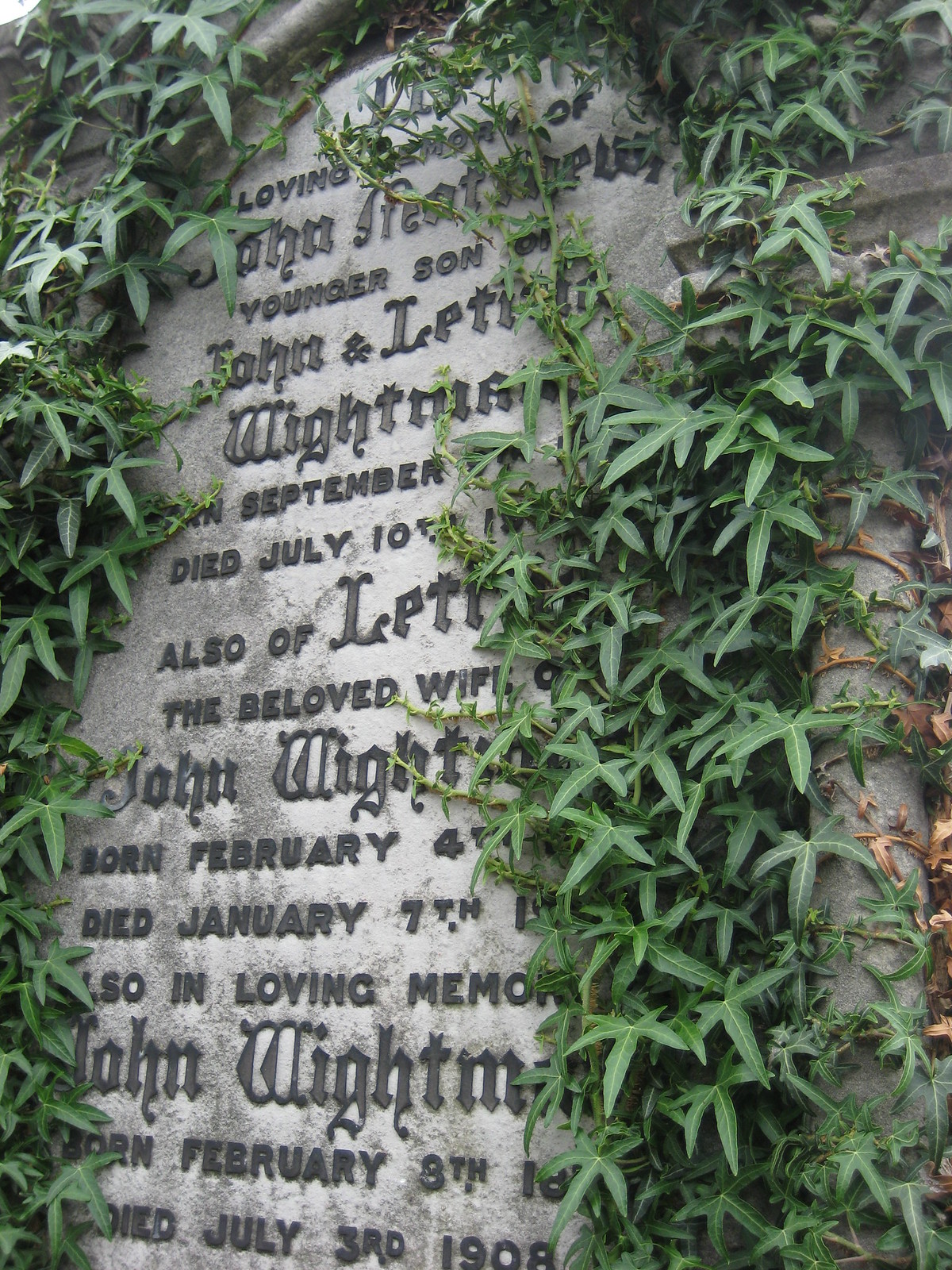The full-color image depicts a stone plaque embedded in a stone wall, partially obscured by overgrown vines and leaves. Despite the vegetation, some inscriptions are still legible. The plaque appears to be a memorial, listing multiple names and dates. The most discernible details include: "In loving memory of John," whose surname is obscured, and references to other individuals named John White and John Whitman. Key dates mentioned are John White, born February 4th and died January 7th, and John Whitman, born January 8th and died July 3rd, 1908. The plaque also notes familial connections, such as John White being the younger son of another John and a reference to the beloved wife of John White. The year 1908 is the most clearly visible date, suggesting the memorials are from a long time ago. Overall, the image illustrates a historical and sentimental record, now partially hidden by nature.